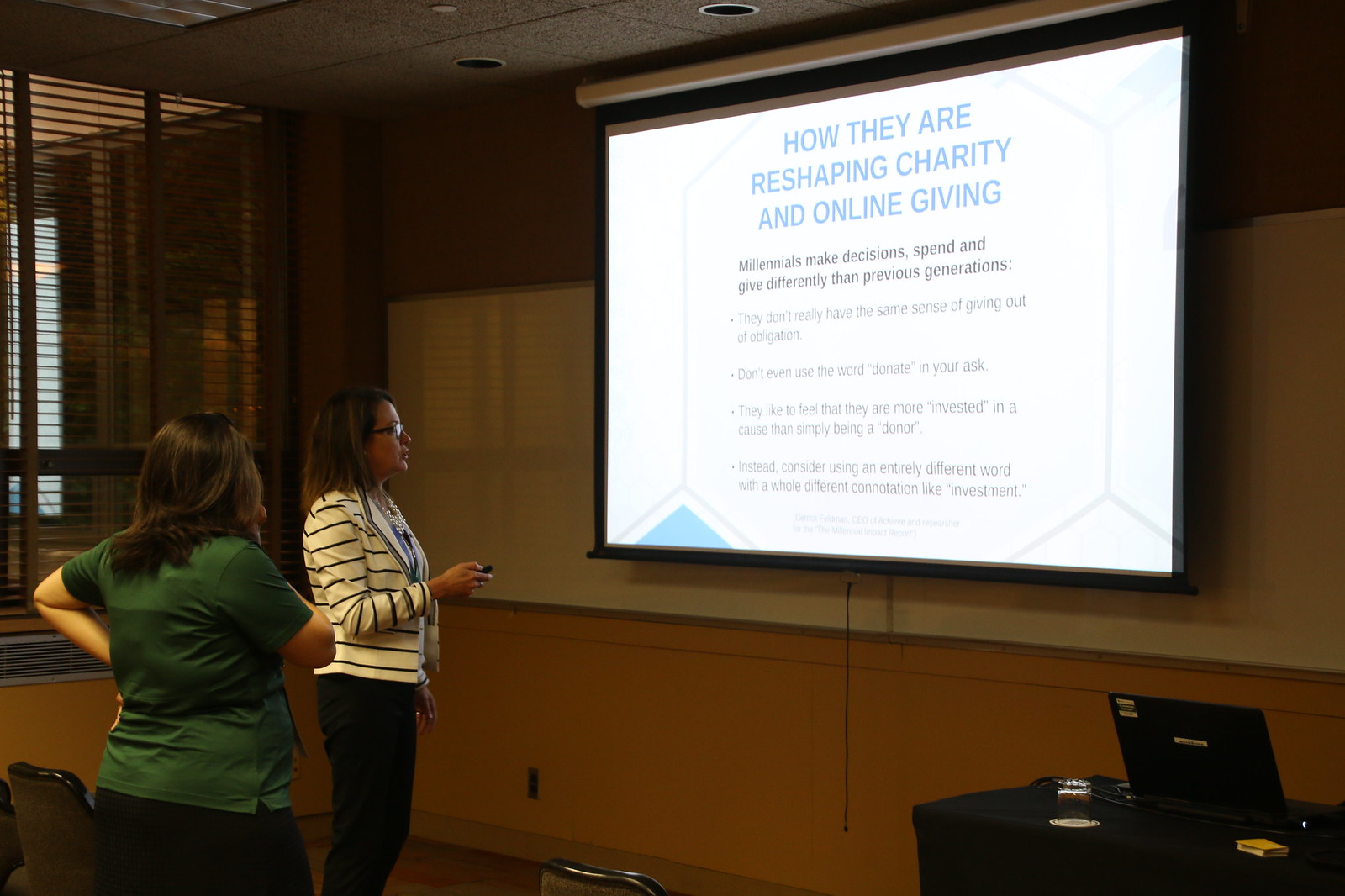In this rectangular photograph, two women are attentively looking at a bright presentation projected onto a screen in a dimly lit office-like room, possibly during a conference or speech. The screen, with a white background and a blue title reading "How They Are Reshaping Charity and Online Giving," displays text in black beneath it that states, "Millennials make decisions, spend, and give differently than previous generations," followed by some bullet points and design elements including a blue triangle on the left and a gray-outlined triangle on the right at the bottom. 

The room has a wall painted in a cream tan color on top and a rusty orange color below a dark chair rail. To the right of the screen is a small black desk with an open laptop and a few other items. The woman on the left, turned away from the camera, wears a green shirt and has dark shoulder-length hair. The woman on the right, who appears to be in her 40s, is holding a clicker to change the slides of the presentation. She has dark, shoulder-length hair, wears glasses, a white jacket with black stripes, and black pants. The background also features some whiteboards and other office equipment, contributing to the professional setting of the scene.